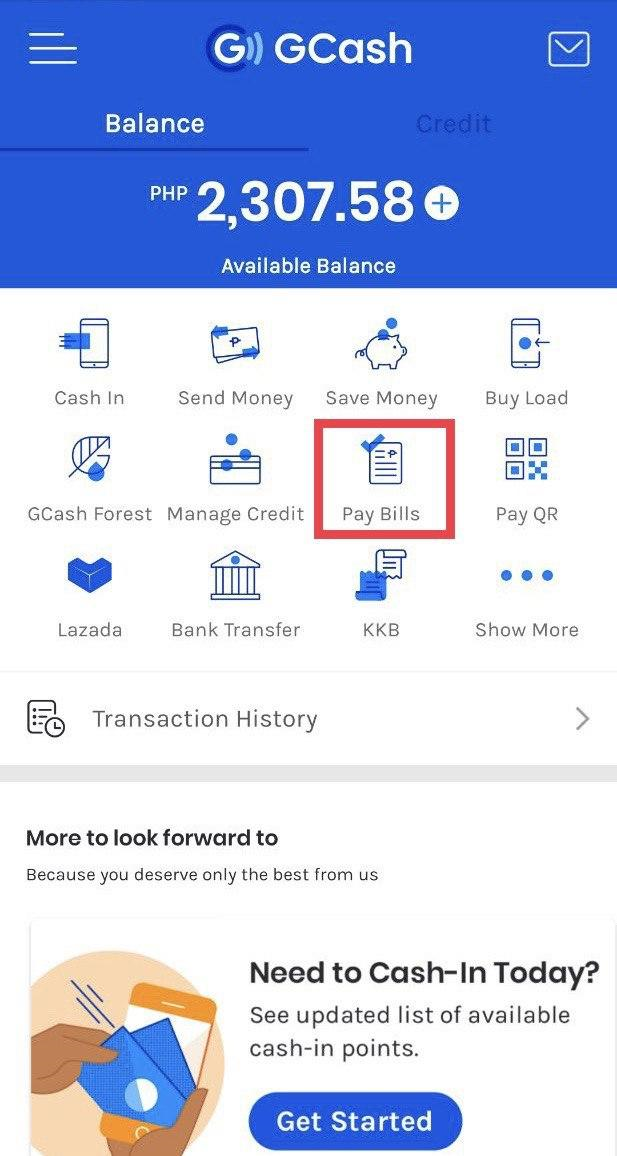This vertical rectangular image features a GCash app interface. The upper section is a horizontal rectangle with a vibrant blue background. At the top, there's a white-font label showcasing the GCash logo; a darker blue circle encloses a capital "G," followed by "GCash" in which the "G" and "C" are capitalized, and "ash" is lowercased. Below this, two options are presented: "Balance," which is currently highlighted, and "Credit," which is darkened. 

Directly beneath this, the text "PHP" is displayed in all capital letters, followed by the amount "2307.58" in large white font, indicating the available balance. Adjacent to the balance, there is a circle with a plus sign inside it. The phrase "Available Balance" is written at the bottom of this blue section, and a small envelope icon is situated in the top right corner.

The lower section has a white background with several words and small icons aligned in rows, all in black text. They read from left to right as follows:
- **First Line**: "Cash In," "Send Money," "Save Money," "Buy Load."
- **Second Line**: "GCash Forest," "Manage Credit," "Pay Bills" (circled in red), "Pay QR."
- **Third Line**: "Lazada," "Bank Transfer," "KKB" (all in caps), "Show More" (with three dots overhead).

Below these options, the text "Transaction History" is followed by a right arrow. Further down, there’s a line that states in black font: "More to look forward to." Directly underneath, in smaller black font, it says: "Because you deserve only the best from us."

Aligned towards the bottom right, it asks in larger black font: "Need to cash in today?" Following this, a smaller text reads: "See updated list of available cash in points." At the very bottom, there's a blue horizontal oval button labeled "Get started."